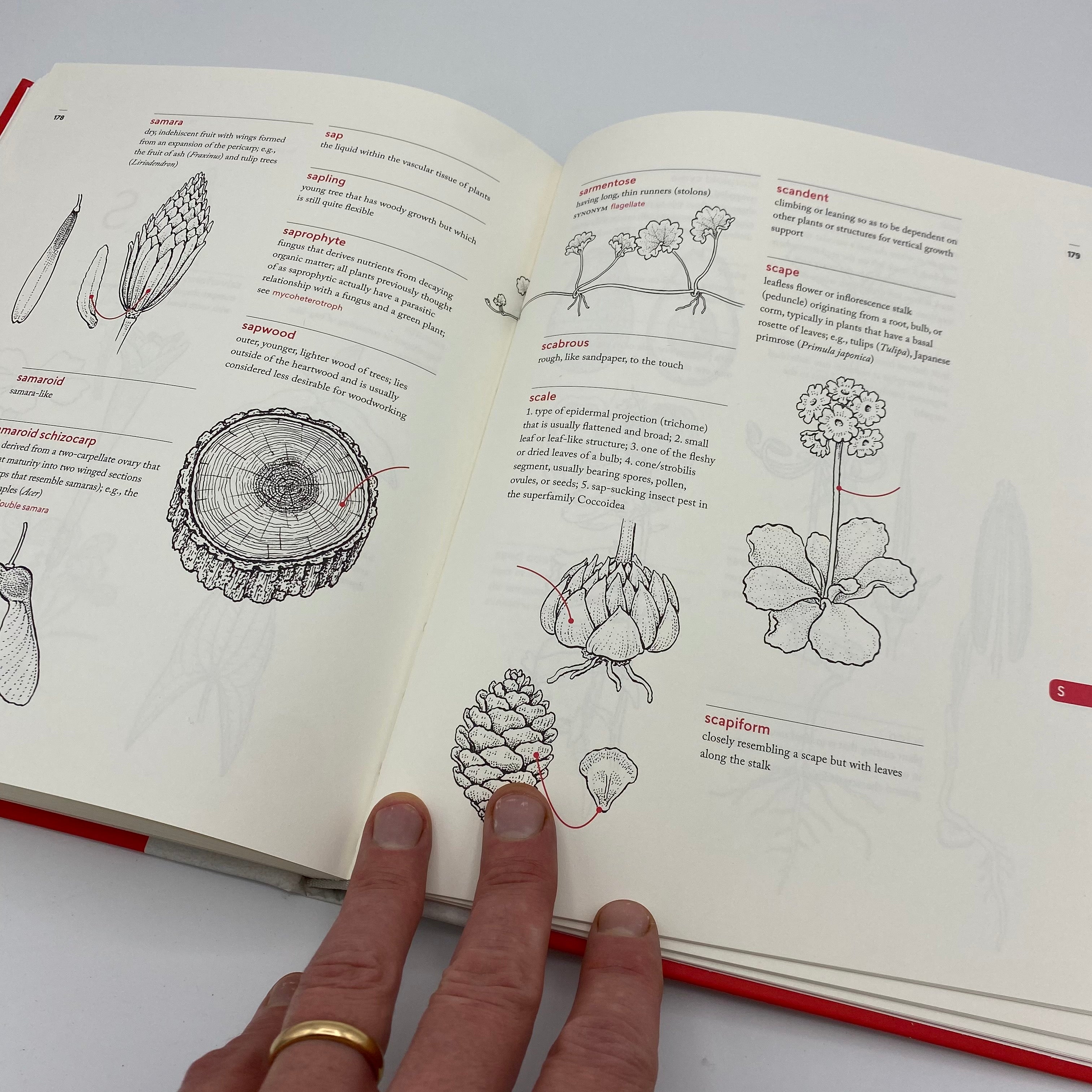A detailed zoomed-in image captures two slanted pages of a book, with the right page extending toward the bottom-right corner of the image and the left page elevated. The book's cover, predominantly red with a small hint of white at the bottom, is partially visible. A hand adorned with a gold wedding band rests gently on the right page, with four fingers in view. The book features botanical illustrations, resembling pages from a science textbook. It includes meticulous drawings of flowers and explanations of their parts and types. One colored diagram highlights a red "scale," described as a type of flat and broad epidermal projection that functions as a small leaf or leaf-like structure. Additionally, the left page showcases an illustrated tree trunk stub. The book is placed on a white surface, providing a clean backdrop for the image.